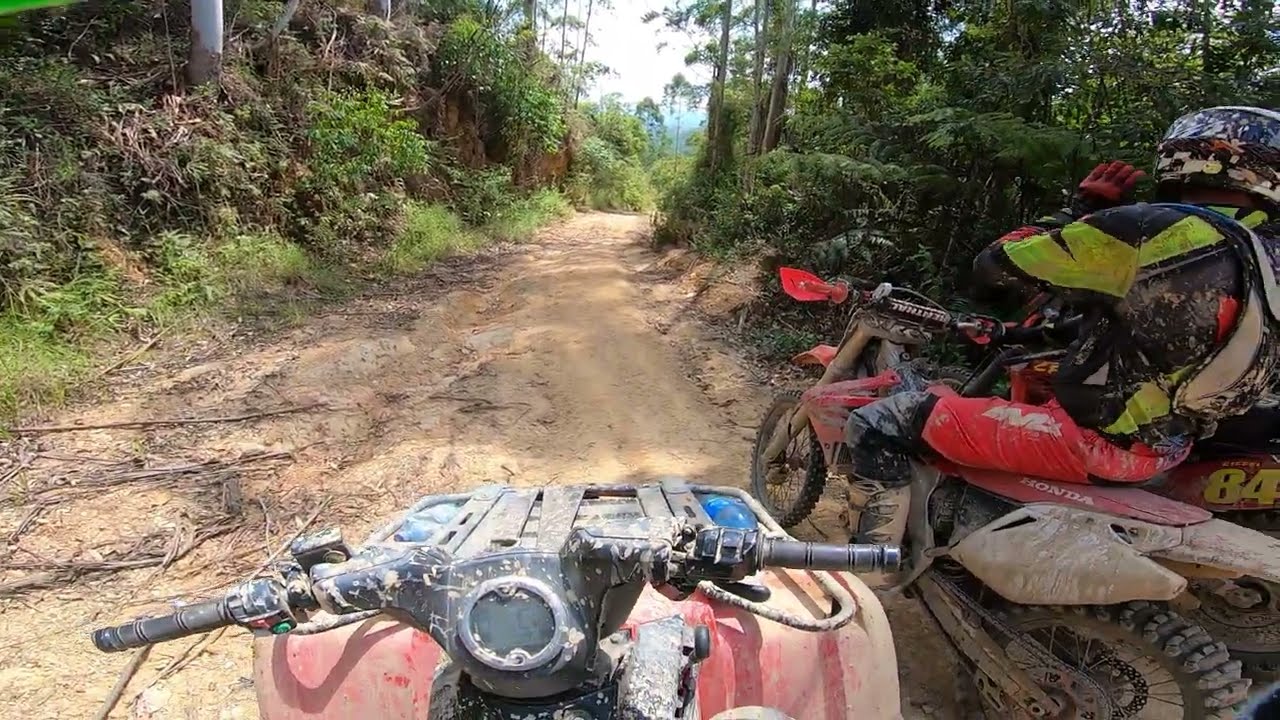The image is a horizontally aligned rectangular picture of two people riding dirt bikes on a muddy dirt path through a dense forest. The path is narrow, flanked by tall, green-leaved trees and some barren branches. The foreground features the front end of a dirt bike, caked in dirt, giving its red bodywork a faded appearance. A closer look reveals the word "Honda" in white on the seat. 

On the right side, a person clad in biking gear—comprising a black and yellow jacket, red pants, and a black helmet—rides another equally muddy Honda dirt bike. The biking outfit is heavily soiled, suggesting they have been riding through muddy terrain for some time. The overall atmosphere suggests it is a bright and partly sunny day, evident by the sparsely clouded white sky peeking through the treetops. The left side of the image shows some branches scattered on the ground, enhancing the rugged appearance of the forest trail. 

The overall scene captures the thrill of off-road biking in a forested area, highlighting the dirt-covered bikes and gear, the intricate details of the surrounding trees, and the riders' adventurous spirit as they navigate the challenging path.